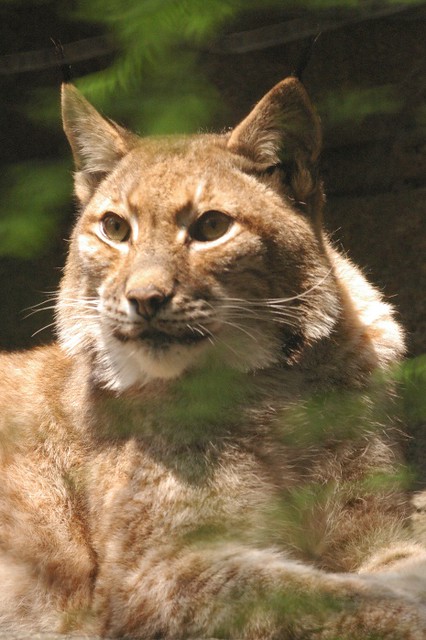The image features a close-up photograph of a large wildcat, resembling a bobcat or possibly a lynx. The cat's fur is a blend of white, brown, tan, and orangey hues, suggesting it is not a domestic feline but a robust, mature wild specimen. Its intense, yellowish-green eyes, along with prominently perched ears and white whiskers, give it a focused and attentive appearance. The background is softly blurred, displaying indistinct shades of green from possible trees or plants and brown from a wall or rock structure. Only the cat's head, chest, and parts of its front legs are visible, highlighting the animal's striking features against the nondescript backdrop.